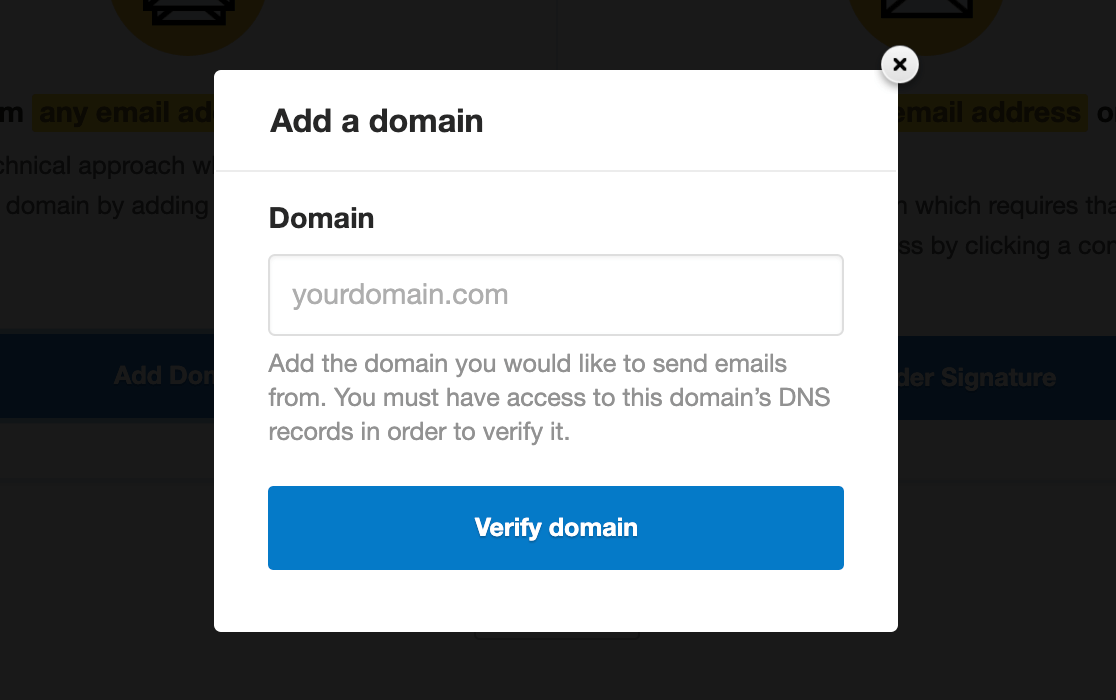The image depicts a website interface where a user is in the process of adding a domain. The background shows white tiles and black text, some of which is highlighted in yellow. At the top left and right corners, there are yellow circles with white envelope icons inside them. A pop-up window is prominently displayed on the screen, featuring a gray circle with a black 'X' in the top right corner for closing it. The pop-up has a white background and a square shape. At the top left of the pop-up, the text "Add a Domain" is written in black. Below that, there is a text box labeled "Domain" where the user can enter the domain name. The instructions below the text box read: "Add the domain you would like to send emails from. You must have access to this domain's DNS records in order to verify it." At the bottom of the pop-up, there is a large blue rectangular button with the text "Verify Domain" centered in white.